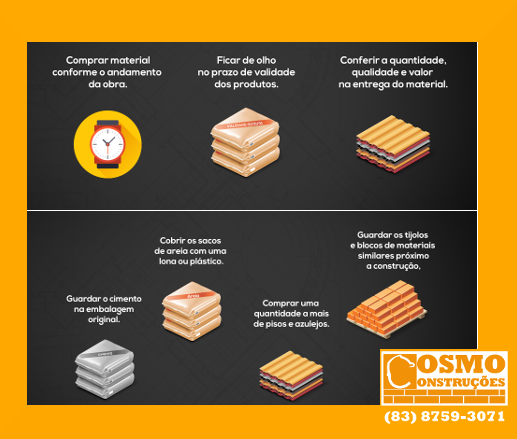The image is a detailed advertisement for a company named Cosmo Construcciones, likely involved in the construction industry, with text in Portuguese. It features a yellow-orange border with a black background, divided into two main sections filled with various items. At the top, there is an illustration of a watch alongside packages that appear to contain construction materials such as bricks, cement, and sand. There is explanatory text over each image: "Comprar material conforme o andamento do obra" next to the watch, "Ficar de olho no prazo de vida dos produtos" next to the packages, and "Conferir a qualidade e valor entrega do material" near other materials. In the bottom right corner, the company logo "Cosmo Construções" is displayed, along with a contact telephone number, 83-8759-3071.